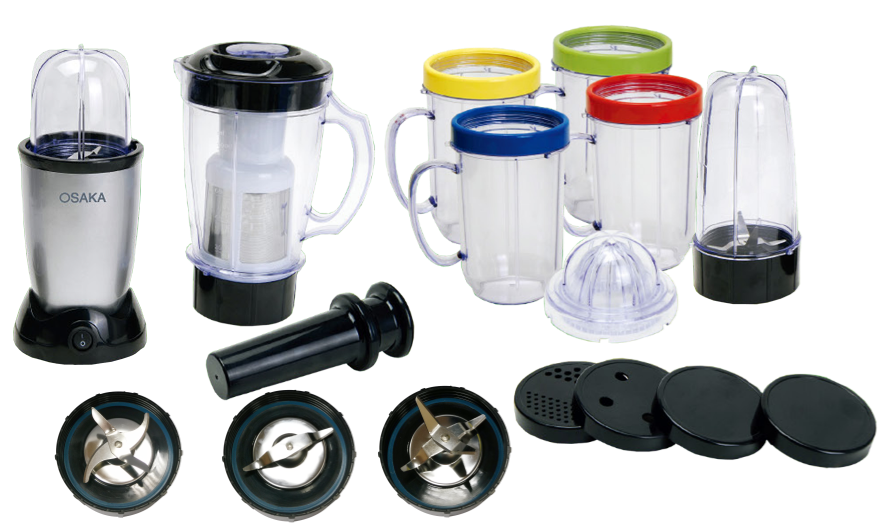This image showcases an extensive array of components for an Osaka multi-attachment blender or food chopper, displayed against a plain white background. On the left-hand side, there's the main blender base featuring an on and off switch, a metal cylindrical body labeled "Osaka," a black base, and a clear plastic top. Adjacent to it is a standard blender pitcher with a black lid and base, a clear middle section, and a white internal cylinder, potentially for blending or processing. Scattered around the base are three types of metallic blades with black rims: one with four straight blades, another with two blades, and a third set with four uniquely shaped blades. A cylindrical black tool, possibly used to push food items down, is located in the center. To the right are four clear cups adorned with colored rims in yellow, green, blue, and red, accompanied by several other attachments, such as lids and replacement parts, some stacked black discs that might be adjustable chopping size regulators. The meticulous arrangement of these parts emphasizes the versatile functionality and comprehensive accessory options of the Osaka blender system.